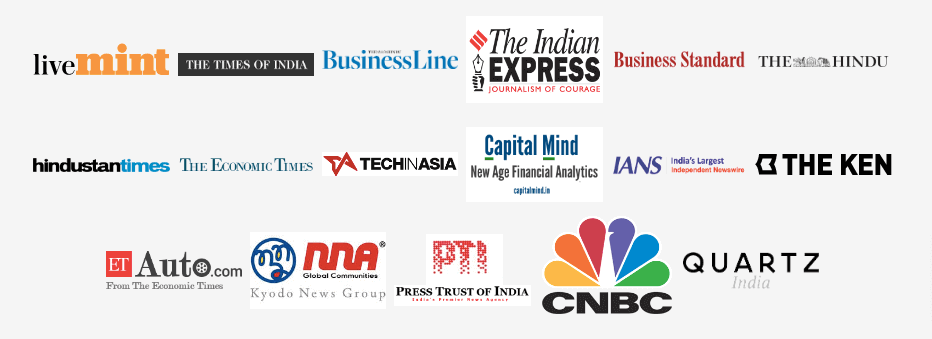This screenshot showcases a collection of prominent company logos and their respective icons, all gathered in a single visual representation. Among the featured entities, the left side highlights Live Mint, with 'Live' displayed in black and 'Mint' in a shade of orange. Also present are the logos of The Times of India, Business Line, The Indian Express, accompanied by its motto "Journalism of Courage", Business Standard, The Hindu, Hindustan Times, and The Economic Times. 

Additionally, tech and finance-focused entities such as Tech in Asia, Capital Mind, and New Age Financial Analytics are included. The display also features IN's, noted as India's largest independent network, along with The Kin and etauto.com, a service from The Economic Times. Other notable inclusions are NNA Global Communities, Kyoto Kodo's news group, The Trust of India, CNBC, and Quartz India. This assortment predominantly represents various significant social media outlets and news organizations operating within India.